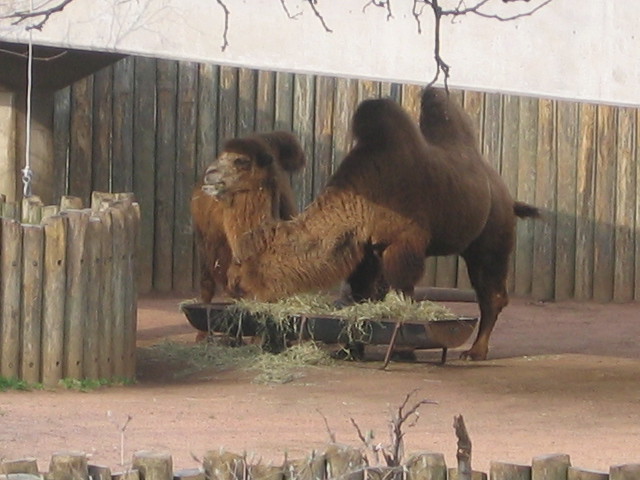This outdoor photograph, rectangular in shape, captures a double-humped camel within a fenced enclosure, likely at a zoo or animal sanctuary. The boundary of the enclosure consists of solid wooden logs forming a sturdy fence. The camel, light brown in color, is kneeling with its front legs in a trough filled with hay, spilling onto the hardscrabble, reddish-brown dirt ground. The camel gazes forward into the distance. Above and around the camel, dead branches hang, suggesting a winter setting. There appears to be another animal partially obscured behind the camel, though its identity is uncertain. A cylindrical wooden container, possibly for water, is visible near the hay trough. The foreground reveals another section of the fence, captured in the sunlight streaming from the center left, casting noticeable shadows across the scene.